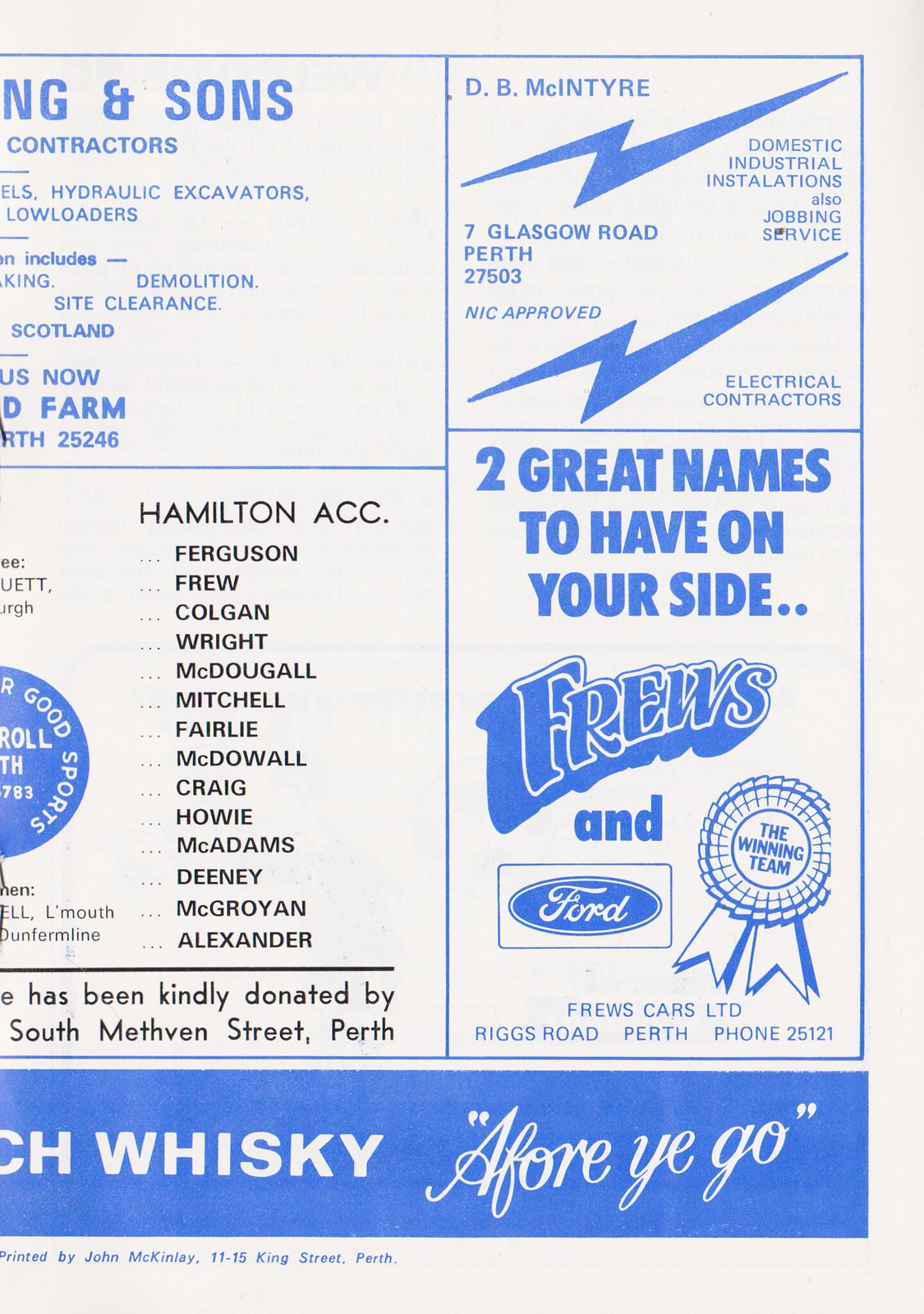The image is a scan of a flyer or pamphlet featuring multiple advertisements arranged into four distinct panels, two on the left and two on the right. The left side of the image is partially cut off, making the text in these panels hard to read. However, on the more visible right side, the top right panel prominently features an advertisement for "DB McIntyre Electrical Contractors," highlighted by two blue lightning bolt logos. This ad includes details such as "Domestic Industrial Installations," "Jobbing Service," "7 Glasgow Road, Perth," "NIC Approved Electrical Contractors," and contact information.

The bottom right panel showcases a promotional segment with the headline "Two Great Names to Have on Your Side" for "Frew Cars Ltd." and "Ford," accompanied by the tagline "The Winning Team." This panel also includes contact details: "Riggs Road, Perth, Phone 25121", with a ribbon-style design element featuring the text "The Winning Team."

The overall color scheme of the image features shades of white, blue, black, and hints of gray, with the various fonts and logos differing in size and style. The advertisements are well spaced within the image, though there is no central focus due to the cutoff sections on the left. The image resembles a piece of printed material such as one you might find in a restaurant or local community space, containing a variety of ad blocks for local businesses.